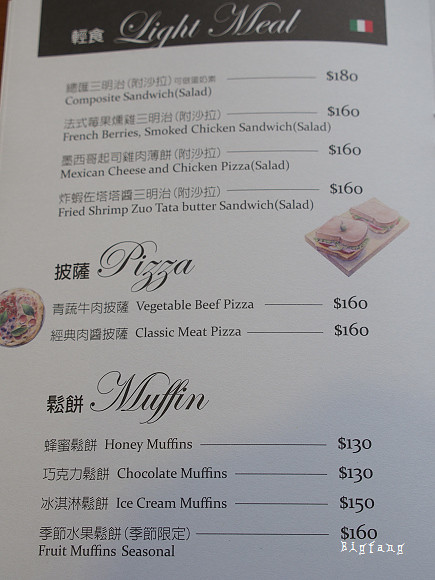The image captures a slightly curved, open menu page, possibly from a Chinese-Italian fusion restaurant, lying on a brown surface that's barely visible in the top left corner. The page, titled "Light Meal," features a distinct layout with Chinese characters alongside an image resembling the Italian flag in a black text box.

At the bottom right of the menu page, a small watermark reads "Big Fang" in white, funky lettering. The menu lists several dishes:

1. Composite Sandwich (Salad) - $180
2. French Berries, Smoked Chicken Sandwich (Salad) - $160
3. Mexican Cheese and Chicken Pizza (Salad) - $160
4. Fried Shrimp Zoua Tata Butter Sandwich (Salad) - $160

Below these items, a small illustration depicts two sandwiches on a wooden board, with the one in the foreground speared by an olive pick. The menu then transitions to pizzas, with a small pizza illustration on the left side of the page:

5. Vegetable Beef Pizza - $160
6. Classic Meat Pizza - $160

The bottom section of the menu lists various muffins:

1. Honey Muffins - $130
2. Chocolate Muffins - $130
3. Ice Cream Muffins - $150
4. Fruit Muffins (Seasonal) - $160

Each muffin item also has corresponding Chinese characters preceding the English description and prices.